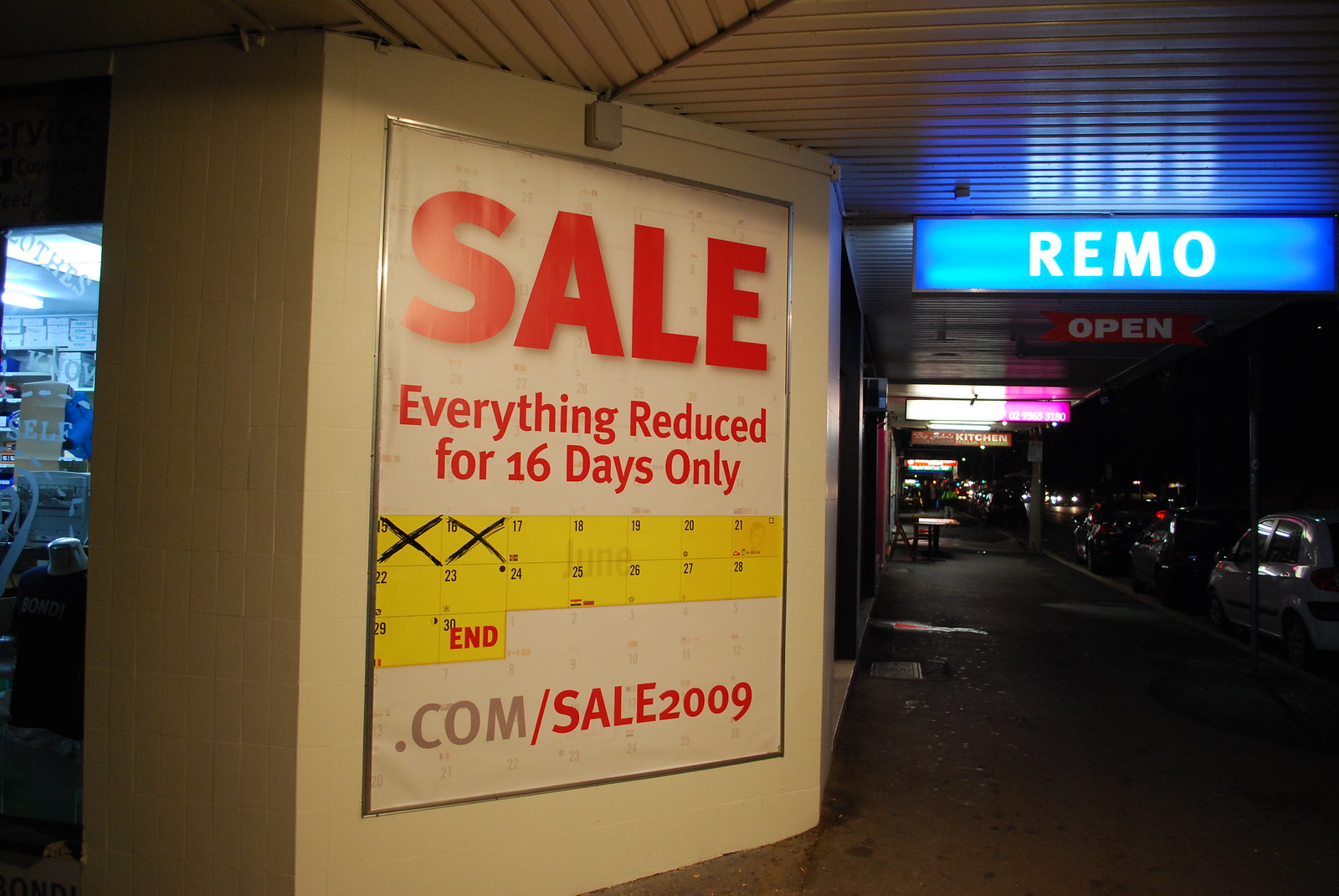This image showcases the dimly lit interior of a shopping mall. To the right side of the image is a parking area illuminated by strip lights, with a prominent blue and white sign that reads "OPEN REMO." On the left side, there is a large advertisement hoarding featuring bold red letters that announce "SALE - EVERYTHING REDUCED FOR 16 DAYS ONLY." Additionally, the hoarding includes a calendar counting down the remaining days of the sale, with a website link "dot com / sale 2009" indicated at the bottom. This sign is strategically positioned to catch the attention of individuals entering the car park.